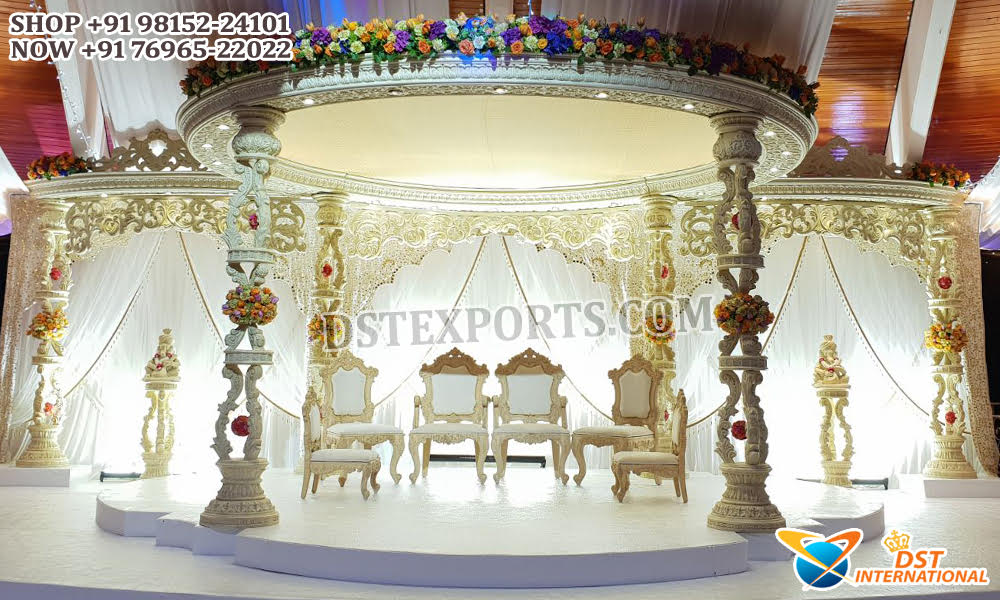The image depicts an AI-generated advertisement likely promoting a venue, possibly located in India, for events such as weddings or receptions. The setting features a large, ornate rotunda adorned with elaborate white and gold designs. In the center of this rotunda, there are six intricately detailed chairs positioned on a raised platform, each with white padding and decorated with lavish ivory or light wood detailing. Flower arrangements embellish the columns that support the rotunda, adding to the luxurious atmosphere. The spacious room is framed by a wooden thatched roof with visible beams, creating an ambiguous sense of being indoors or outdoors. The advertisement includes a call-to-action with non-American phone numbers at the top, indicating international accessibility. The bottom left corner displays the logo "DST International" with imagery featuring a crown and a planet encircled by red and gold rings. The prominent emphasis on white, gold, and floral elements underscores the venue's opulence and suitability for grand celebrations.